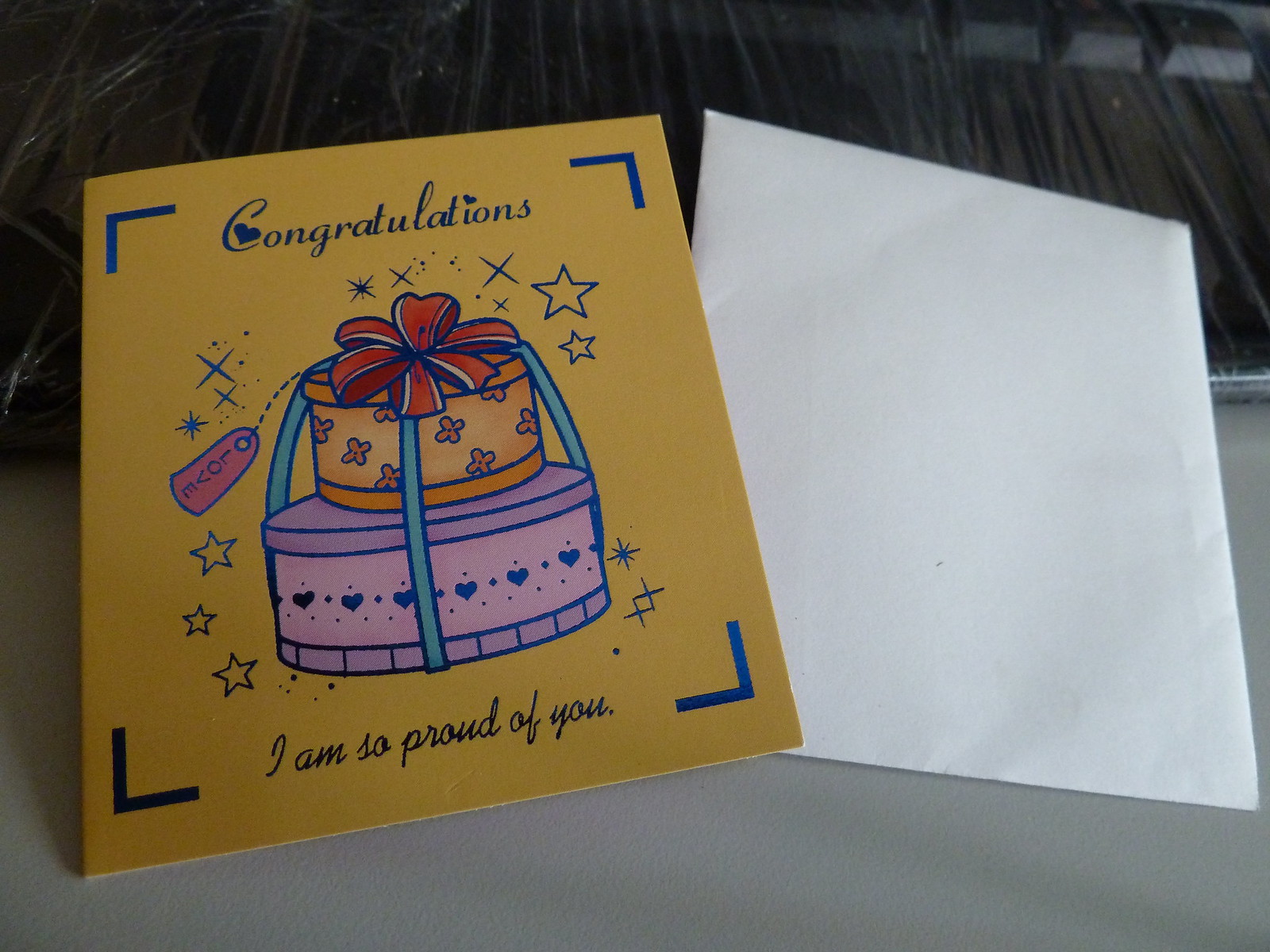In the image, there is a yellow congratulations card and a white blank envelope resting on a gray surface or possibly a plastic-wrapped keyboard. The card, positioned on the left, has a cheerful yellow background with four blue lines on the corners. At the top, in blue cursive, it reads "Congratulations," with a heart integrated into the letter "C." The center of the card features a brightly colored, two-layer cake - the top layer is yellow with an orange cross pattern resembling X's, and the bottom layer is purple decorated with hearts. A blue string runs the length of the cake, tied in a red bow at the top, and a pink tag on the cake reads "love" in blue letters. There are also little stars around the cake for additional decoration. At the bottom of the card, it says "I am so proud of you" in blue cursive. To the right of the card lies a plain white envelope, suggesting that this card may soon be sent or given to someone special.